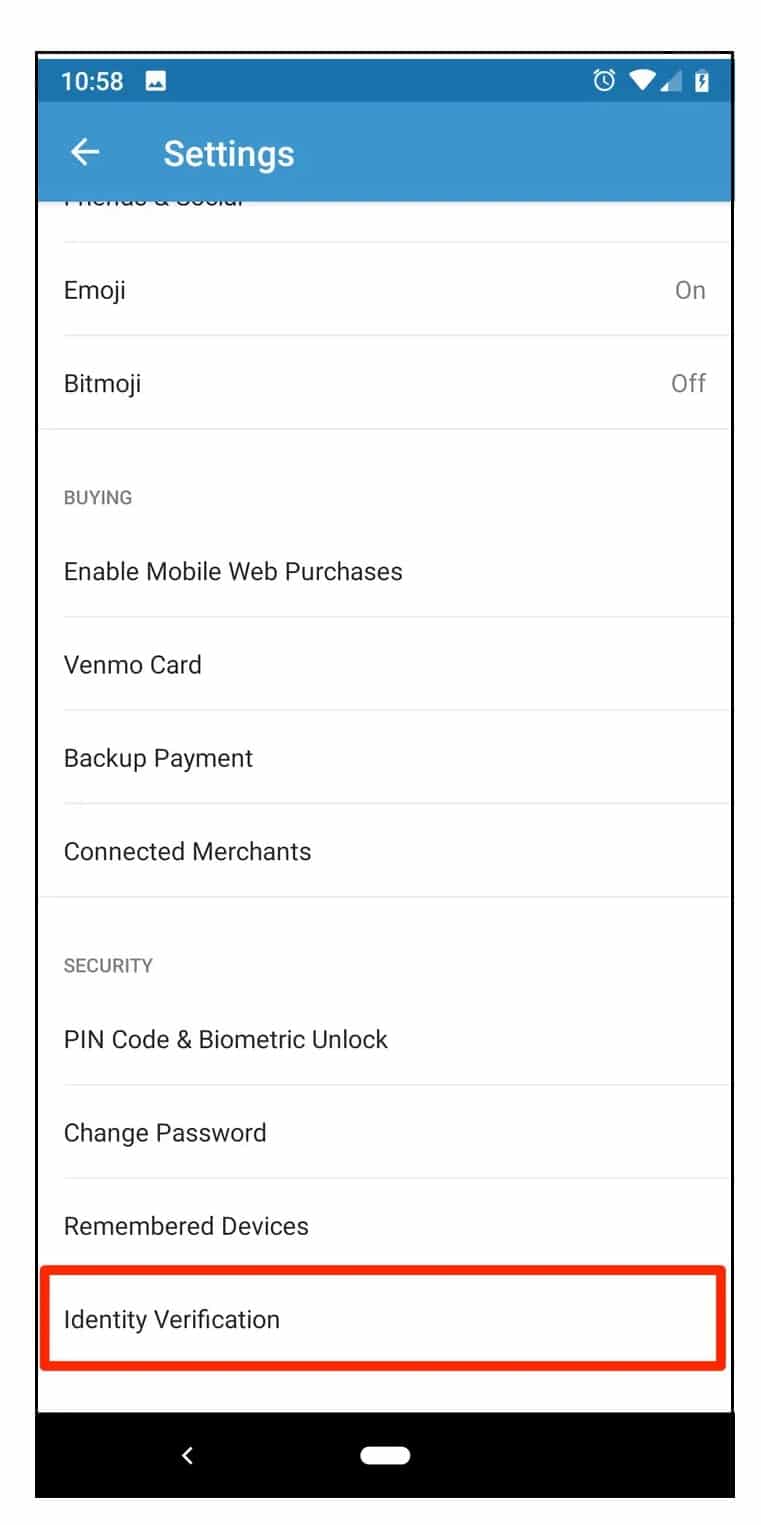The screenshot depicts a settings interface, likely from a mobile device or application. At the very top left corner of the image, the device's time is displayed as 10:58. On the top right corner, a series of icons are visible: an alarm icon, a Wi-Fi icon, a data connection icon, and a battery icon.

Directly beneath these icons, there is a prominent blue banner with the word "Settings" aligned to the left. Under this banner, several settings options are listed in a structured format:

- "Emoji" appears on the left with the status "On" indicated on the right.
- "Bitmoji" follows, with the status "Off" on the right.
- "Buying" is listed next, leading into more detailed options below it:
  - "Enable mobile web purchases"
  - "Venmo card"
  - "Backup payment"
  - "Connecting merchants"

The section continues with security-related settings:
- "Security" heading
  - "PIN code"
  - "Biometric unlock"
  - "Change password"
  - "Remember devices"
  - "Identity verification"

Each term and status are clearly delineated, making it easy to navigate and understand the various options available for configuration.